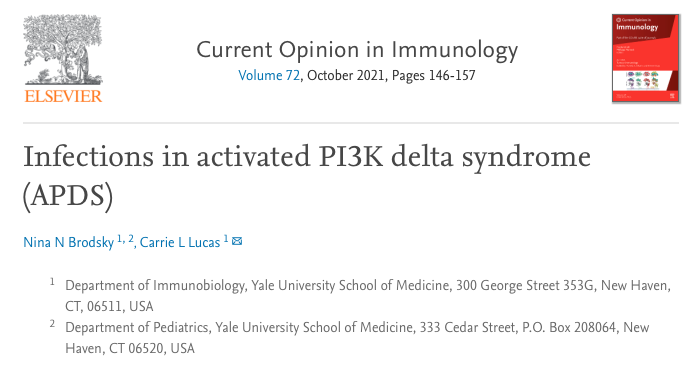This is a screenshot of a page from a journal article database, specifically from Elsevier. In the top left corner, the Elsevier logo appears, featuring a black and white pencil graphic of a tree. The main focus of the page is an article titled "Current Opinion in Immunology," published in Volume 72, October 2021, spanning pages 146 to 157. To the right of this title is an image of a book titled "Immunology." The book has a red cover with darker red accents and features a white section with colorful diagrams likely depicting microorganisms.

Below the book image, the specific article title "Infections and Activated PI 3K Delta Syndrome (APDS)" is displayed. The authors of the article are Nina A. Brodsky and Carrie L. Lucas. At the bottom of the page, two citations are listed vertically. The webpage has a simple, white background with straightforward formatting, characteristic of an academic journal website.